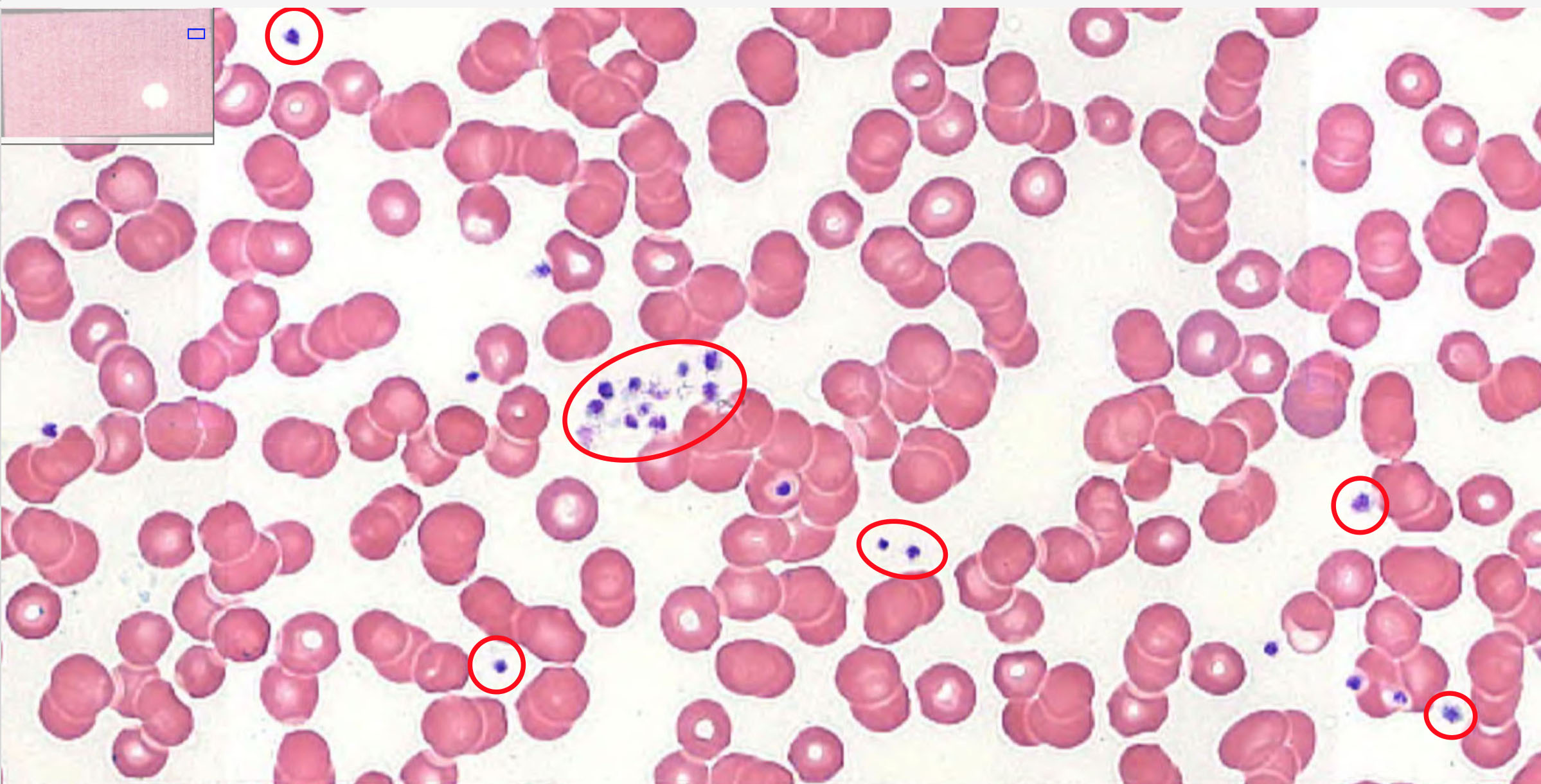The image appears to be a view under a microscope, dominated by various geometric shapes, primarily circular and hexagonal, which are filled with pink color and cover the entire visual field. These shapes vary in their arrangement; some touch each other, while others are separated by white gaps. In the gaps, there are small blue dots, some of which are isolated, while others form clusters. Certain blue dots are circled in red, highlighting them against the background. Notably, in the center upper-left area, there's a prominent red circle encompassing a cluster of several blue dots. Additionally, the top left-hand corner of the image features a pink rectangle containing a smaller blue rectangle in its top right corner, and a white circle towards its lower side. The overall background of the image is white, enhancing the visibility of the colored elements.